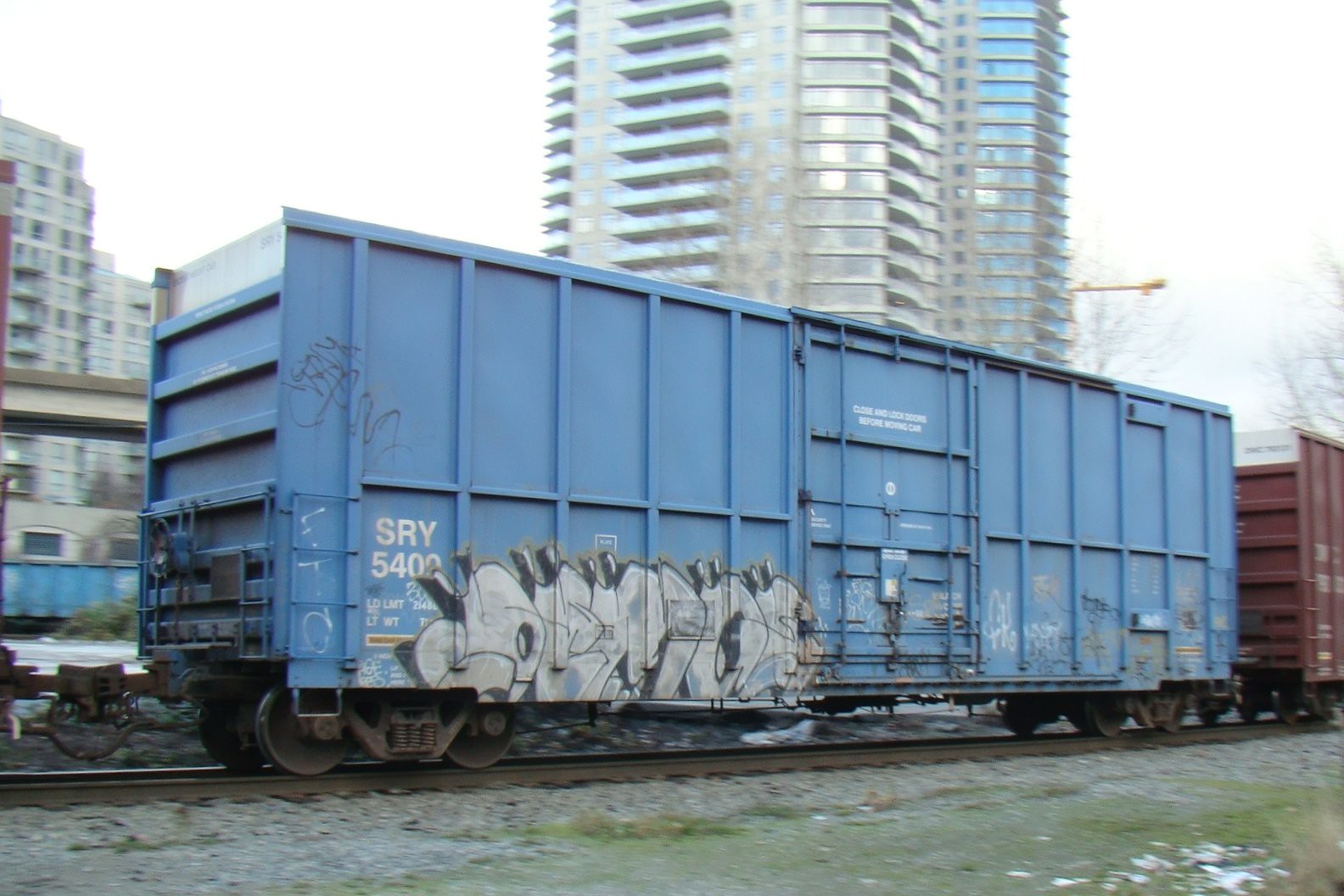This outdoor daytime photograph captures a cityscape under gray, cloudy skies, suggesting a winter setting. Dominating the image is a blue, plug door-type railroad freight boxcar, labeled with white text "SRY 5400" and adorned with white graffiti on the lower left side. The boxcar appears slightly blurred, indicating movement along rusty brown tracks. Adjacent to it, the rear edge of a brown boxcar is visible. The grassy foreground contrasts with a backdrop of a tall, silver and gray multi-story apartment building, which extends beyond the frame's top edge. The background also includes leafless tree tops to the right, reinforcing the wintry atmosphere.